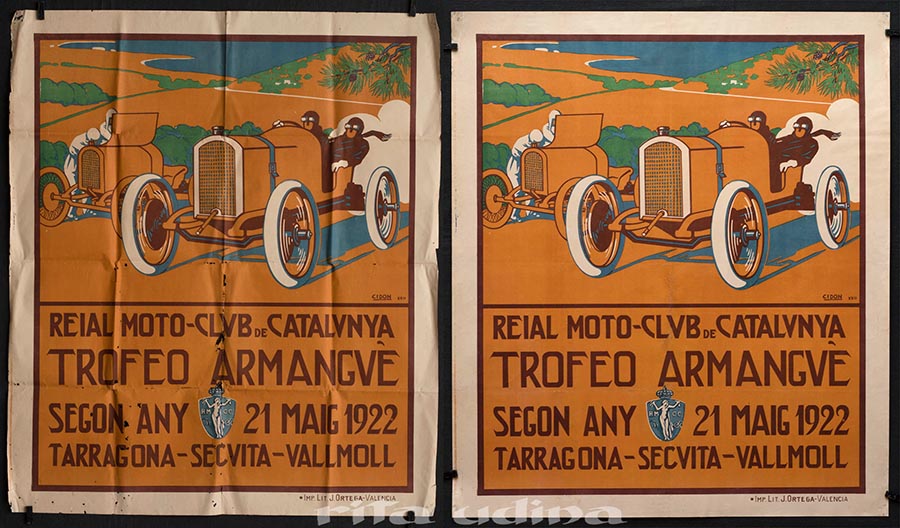The image depicts two identical posters side-by-side, showing signs of wear as if they have been exposed for several days. The poster on the left is particularly tattered and wrinkled, while the one on the right remains crisp and clean. Both posters feature an old-fashioned car with large white wheels and a prominent grille, driven by two men in black attire wearing goggles. Behind the car on the far side, another car with its hood up is visible, displaying the silhouettes of two men working on it. The backdrop is an orange landscape with green patches and what looks like white clouds of smoke or exhaust. The bottom half of the posters is occupied by black text in Italian, reading "Real Moto Club de Catalonia" and "Trofeo Armangov", along with a date: 21st March 1922. The scene captures an open field, likely a race setting, possibly in Tarragona.